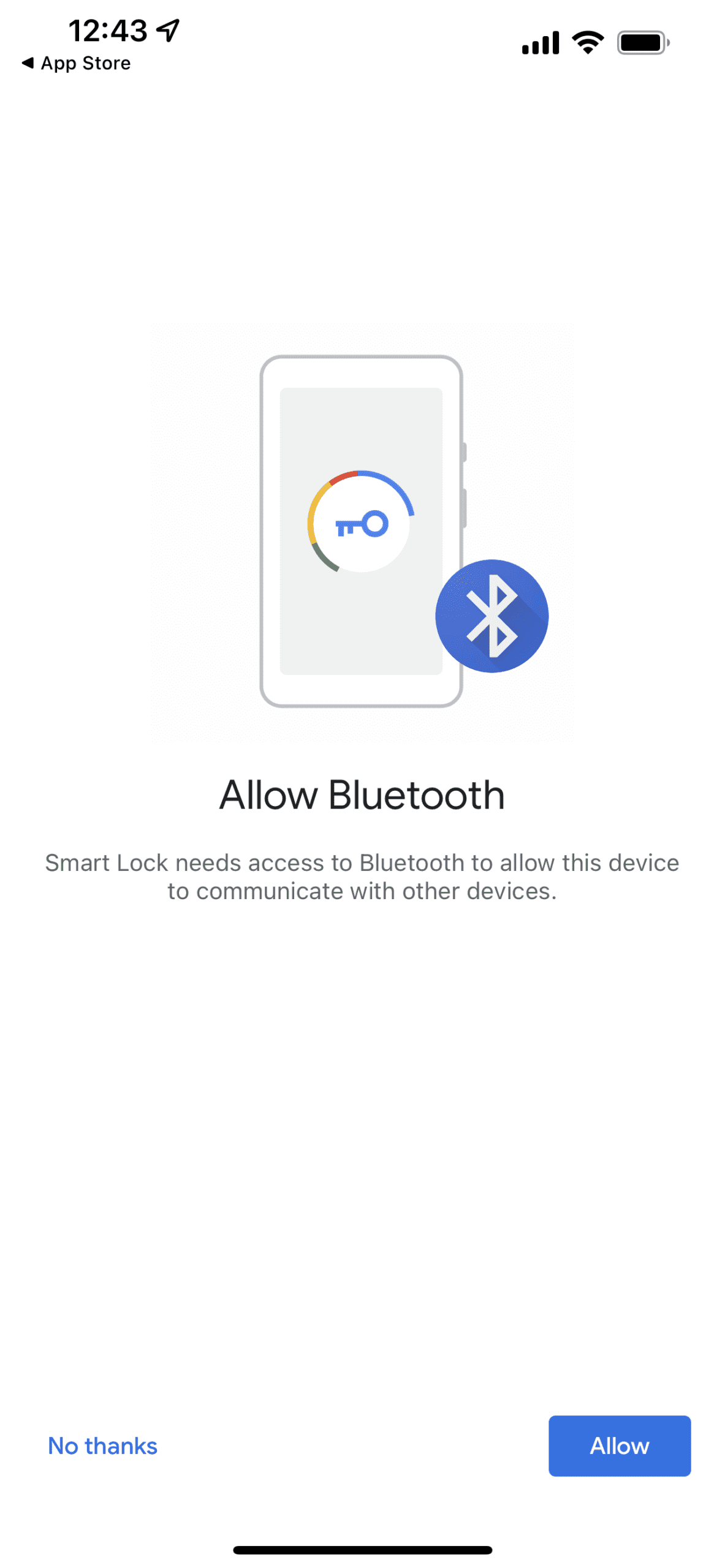This screenshot shows a pop-up notification on a smartphone screen. At the center of the screen, there is a circular icon featuring a blue key, symbolizing security, with a small Bluetooth icon located at the bottom right of the circle. Beneath this icon, bold text reads "Allow Bluetooth." Further down, explanatory text states, "Smart Lock needs to access Bluetooth to allow this device to communicate with other devices."

At the bottom of the notification, on the left, the option "No Thanks" is presented in blue text. On the right side, a solid blue box contains the word "Allow." The background of the pop-up is white.

At the top left corner of the screen, the phone's clock displays the time as 12:43. In the top right corner, icons for signal strength, Wi-Fi connectivity, and battery level are visible.